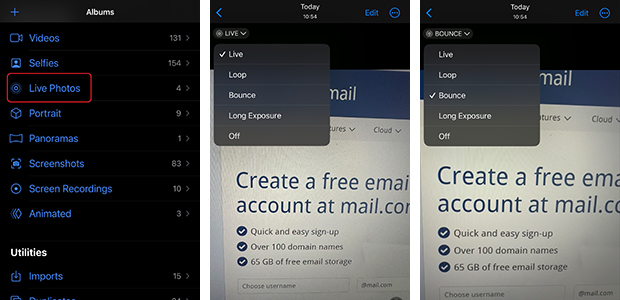The collage of three snapshots showcases different views of the Photos app on an iPhone. 

In the first image, the main screen of the Photos app is displayed, highlighting various album categories: 131 videos, 154 selfies, 4 live photos, 9 portraits, 1 panorama, 83 screenshots, 10 screen recordings, 3 animated photos, and 15 imported items grouped under utilities.

The second snapshot zooms in on one photo, revealing live photo editing options under the 'Today' tab, timestamped at 10:54 AM. The options available for the live photo include 'Live,' 'Loop,' 'Bounce,' and 'Long Exposure.' Additionally, there is a small ad banner at the top promoting the creation of a free email account at mail.com, boasting quick and easy signup, over 100 domain names, and 64 GB of free email storage. The 'Live' option is selected in this image.

In the third and final snapshot, the focus shifts to the same photo, now with the 'Bounce' effect selected, demonstrating a dynamic change in how the live photo is displayed.